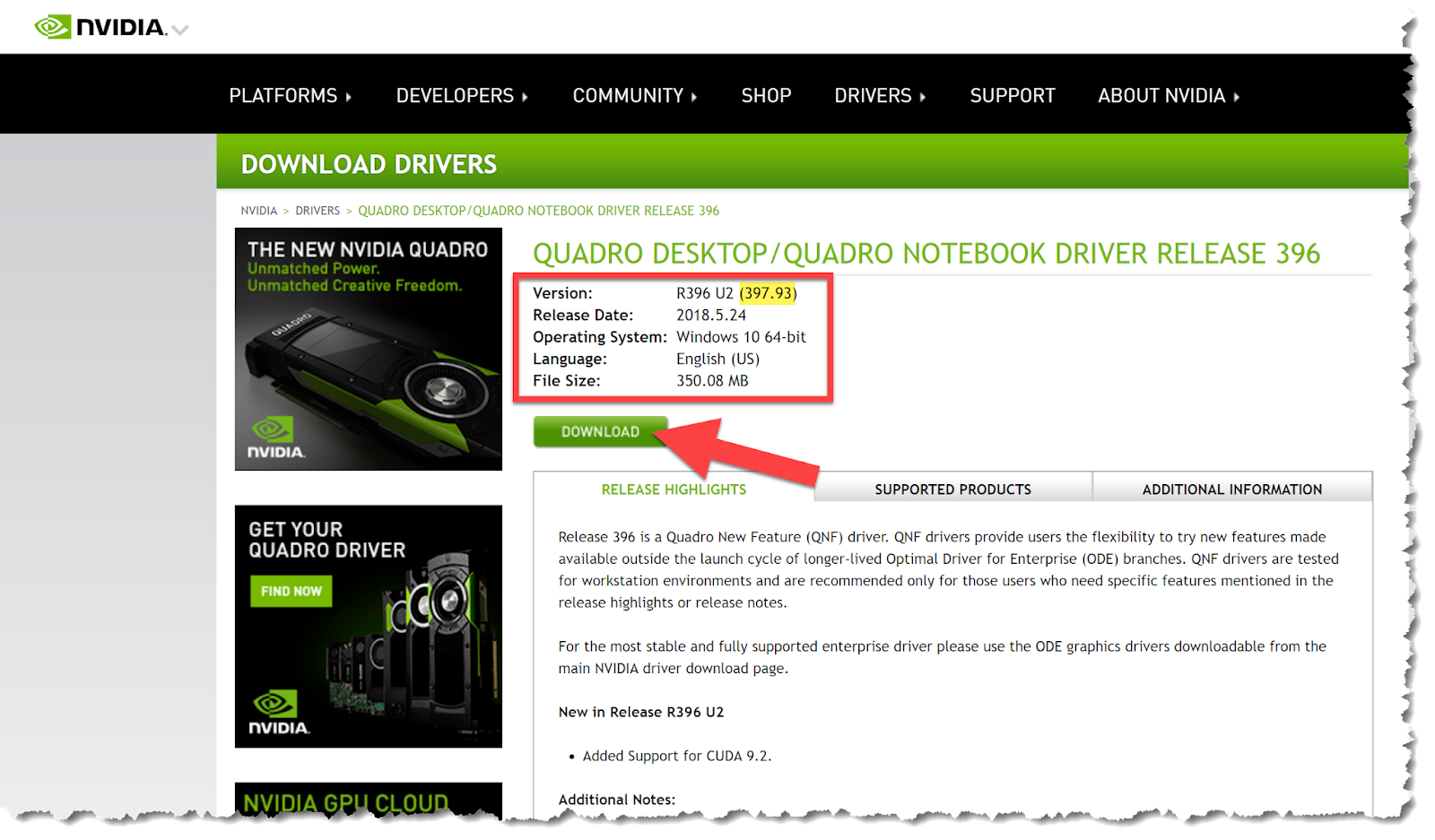From the NVIDIA website, the image features a structured layout with a black navigation bar at the top containing the following options: Platforms, Developers, Community, Shop, Drivers, Support, and About NVIDIA. Beneath this, a green banner prominently displays the text "Download Drivers."

Centered within the image is a promotional section for the new NVIDIA Quadro graphics card, showcasing its tagline: "Unmatched Power, Unmatched Creative Freedom." The centerpiece is a sleek black graphics card with green accents. To the right of the card, detailed driver release information is presented: "Quadro Desktop / Quadro Notebook Driver Release 396." A highlighted red box indicates the version as "R396U2" with a parenthetical note "397.93" and a highlighted yellow area details the release date as "2018.5.2.24." Additional specifications include compatibility with "Windows 10 64-bit" and the language set to "English US." The file size is noted as "350.08 MB."

A prominent green "Download" button with a red arrow pointing towards it draws attention for immediate action. Below, the interface features three tabs: "Release Highlights," "Supported Products," and "Additional Information," with "Release Highlights" being the active tab shown, displaying extensive text content. 

To the left sidebar, there is another promotional image with the text "Get Your Quadro Power, Find Now," showcasing multiple graphics cards to emphasize the product lineup.